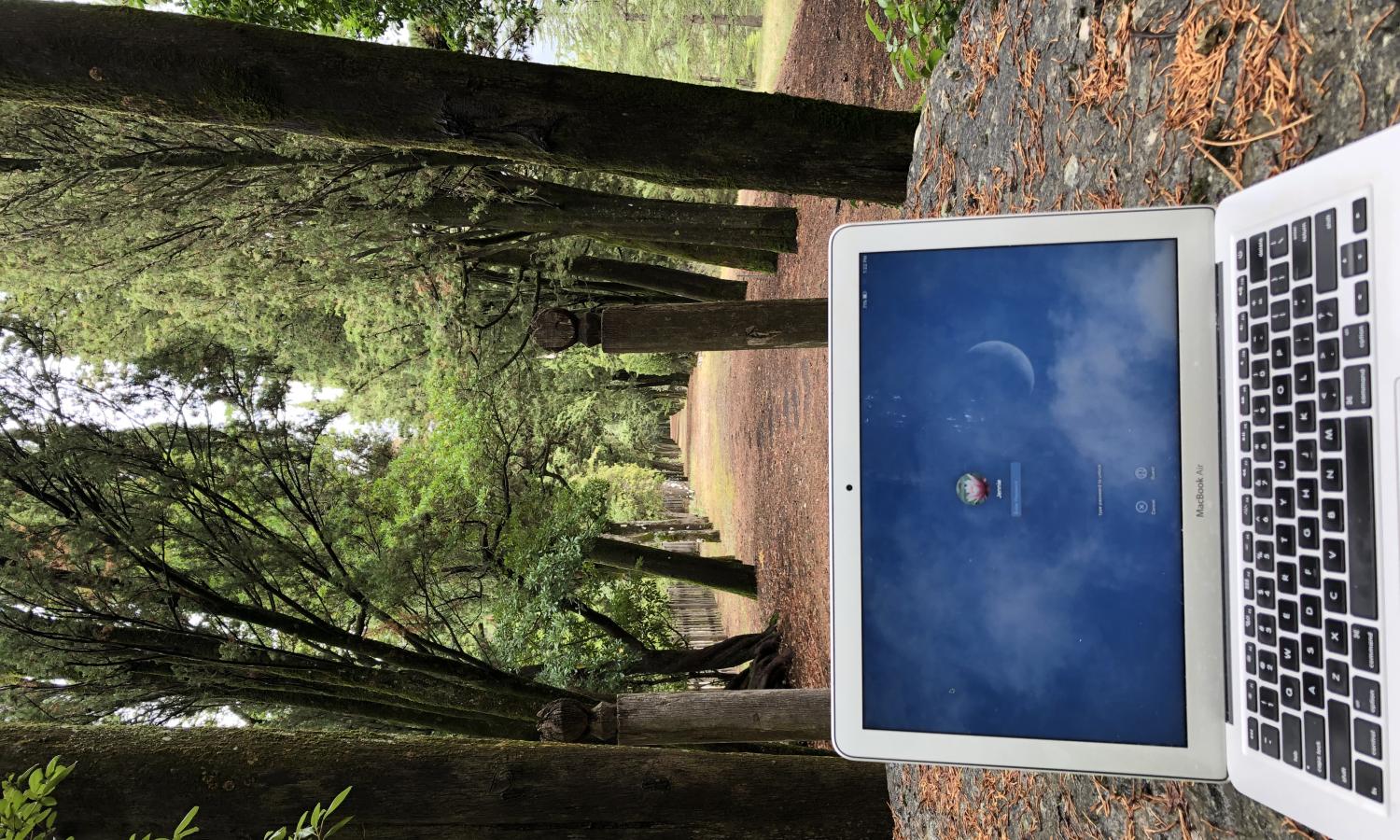In this unusually oriented photograph taken from the perspective of someone using the laptop, the entire image is flipped on its left side, creating a horizontal view of a serene forest scene. On the right side of the image lies a silver Chromebook laptop, distinctly characterized by its black keys and an activated screen displaying a blue background. The left side of the image is dominated by a dense forest with green trees, a mix of pine and possibly elm, leading up to a centrally located pathway. This light brown or golden trail, carpeted with dead leaves, branches, and some dead grass, cuts through the woods and extends to where the laptop is resting. Contrary to appearing directly on the dirt surface, the laptop seems to be placed on a stone table scattered with some leaves, harmoniously blending with the natural surroundings. The overall impression is that of a real-life photo, potentially intended for social media, capturing a moment of digital interaction amidst the natural world.